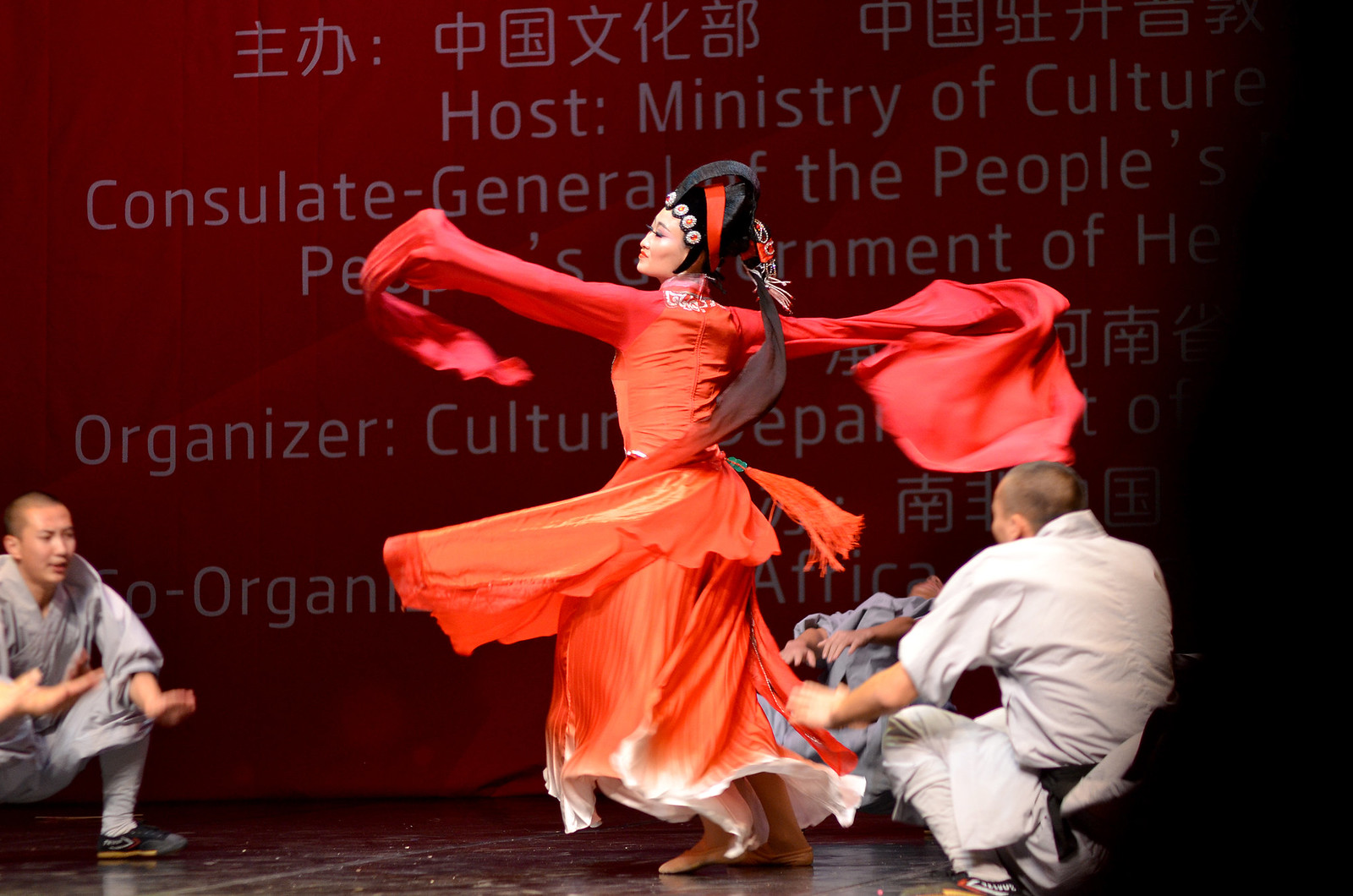In this captivating image, an Asian woman is performing a dynamic, twirling dance in the center of the scene, surrounded by men kneeled down in what appear to be karate uniforms. She is dressed in an elegant, long-flowing orange dress with white at the bottom, which flares dramatically as she spins. Her arms are outstretched, causing the dress to billow out, creating a sense of movement. The dress features red sleeves that extend well beyond her hands, adding to the visual spectacle. The woman sports an ornate black hat adorned with orange and embellished with long, flowing cloth that spirals around her body. 

Her hair, dark and long, cascades down her back and past her waist. Despite her body facing away, she has turned her head sharply to the left, her expression focused. 

To her left and behind her, two men in gray suits—one somewhat blurry—are kneeling and looking towards her feet. The man directly behind her appears to be looking down while holding his hands out in front. Additionally, another martial artist kneels on the opposite side, seemingly ready to engage, adding a sense of imminent action.

In the background, a large banner displays Chinese characters and partially visible English text that reads "Host Ministry of Culture, Consulate General of the People, Organizer, Culture," though much of it is obscured by the performers and shadows. The setting appears to be an indoor venue with a solid floor, contributing to the overall dramatic and kinetic atmosphere of the scene.